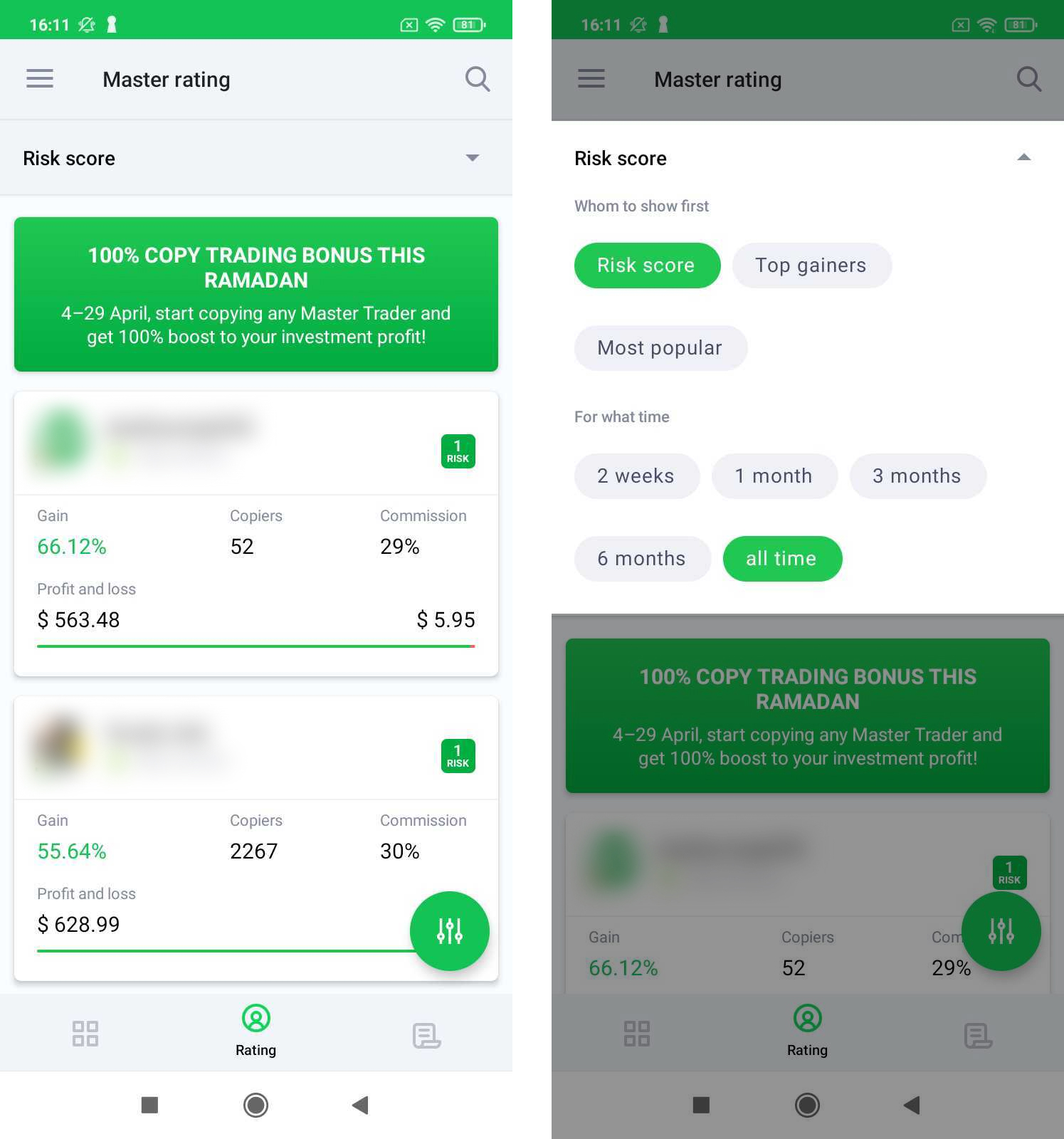The image features two vertically aligned phone screenshots, predominantly white and green with some gray elements. Both screenshots display the time as 16:11 in the upper left-hand corner, and in the upper right-hand corner, there are Wi-Fi and battery symbols, each showing 61% battery life.

At the top of the screenshots, there's a header with a dropdown list labeled "Master Rating" and a search bar. Underneath, the "Risk Score" option is selected, providing detailed information. A green box with white text prominently displays a promotional message: "100% copy trading bonus this Ramadan before 29 April. Start copying any master trader and get a 100% boost to your investment profit."

Following this message, a section lists various risk scores and metrics:
1. A box labeled "Risk 1" includes:
   - Gain: 66.12%
   - Copiers: 52%
   - Commission: 29%
   - Profit and Loss: $563.48 
   - Total Commission: $5.95

2. Another entry shows:
   - Gain: 55.64%
   - Copiers: 2,267
   - Commission: 30%
   - Profit and Loss: $628.99

A filter at the bottom of the screenshots shows options to sort by "Risk Score," "Top Gainers," and "Most Popular." The "All Time" filter is selected by default, as opposed to "Two Weeks," "One Month," "Three Months," and "Six Months." This filter is currently set to display information for all time. 

In summary, the detailed attributes of each "Risk Score" align with the promotion, ensuring users have comprehensive data to incentivize trading activities.